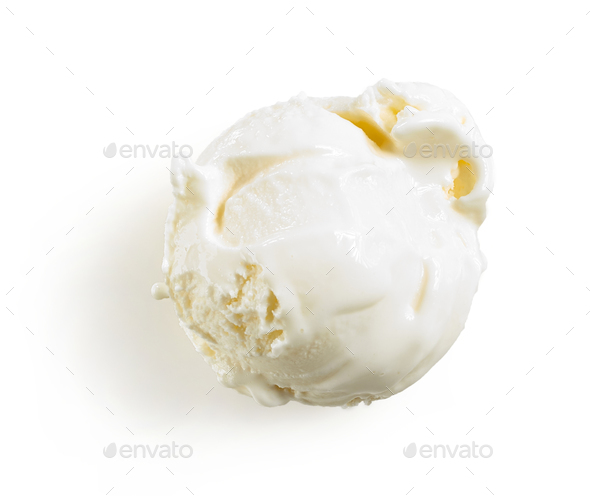The image features a scoop of vanilla ice cream, white in color, centered against a solid white background. The ice cream scoop, though mostly round, has an uneven texture with a noticeable larger cut on the top left and minor cuts scattered across. These cuts reveal a creamy yellow color beneath. The bottom left side of the scoop appears more uneven, while the bottom right side is smoother. A shadow of the scoop is cast on the lower left corner of the image. Surrounding the ice cream, the background contains the word "Envato" in lowercase gray letters, interspersed with faint gray dashed lines forming a diamond pattern, serving as a watermark. There are no additional texts or symbols other than this watermark throughout the image.